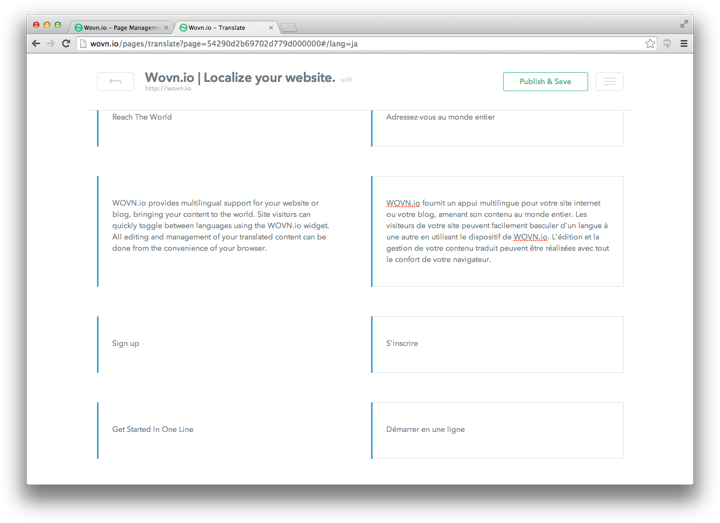Screenshot of a browser window using Chrome, identifiable by the red, yellow, and green dots located on the upper left-hand corner of the gray browser bar. The currently active tab is labeled "WOVN.IO Page Manager" in bold black text, distinguished by a green icon next to the "W" in "WOVN." Adjacent to it is another tab titled "WOVN.IO Translate," also accompanied by the same green icon.

Directly below the tabs is the URL bar containing navigation buttons, including a reload button and left-right arrow icons on the left side. The primary content of the page is displayed below the URL bar against a white background. It prominently features the text "WOVN.IO Localize Your Website" in bold black font, with the website's URL visible directly beneath that.

Further down, a section with a thin blue vertical border on the left and right edges presents the message, "Reach the World." This section explains that "WOVN.IO provides multilingual support for your website or blog." 

In the upper right-hand corner of the page is a blue-outlined button labeled "Publish and Save" in blue text. Additionally, the information on the left side of the page is translated into French on the right side, indicating WOVN.IO's capability to offer multilingual support.